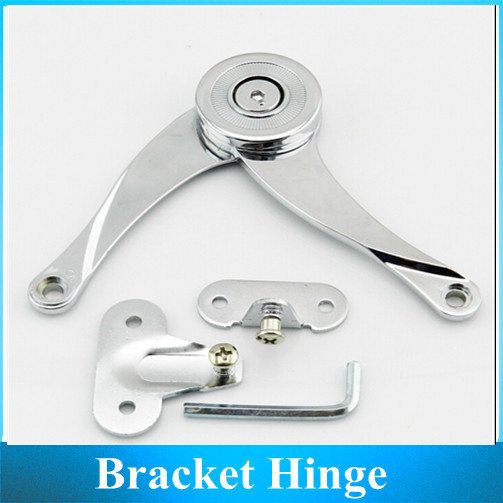This image depicts a shiny silver bracket hinge prominently centered against a solid light gray background with a blue outline. The hinge, shaped like an upside-down 'V' with a thicker circular top, extends into two wavy arms, each ending in small cutout circles. Directly beneath the hinge are additional components: a flat piece with holes on the left and right sides, and two screws—one going through the front and another perpendicular to it from the top. Adjacent to these elements is a thin, L-shaped metal piece. At the bottom of the image, "BRACKET HINGE" is clearly spelled out in white letters against a turquoise blue rectangular background.